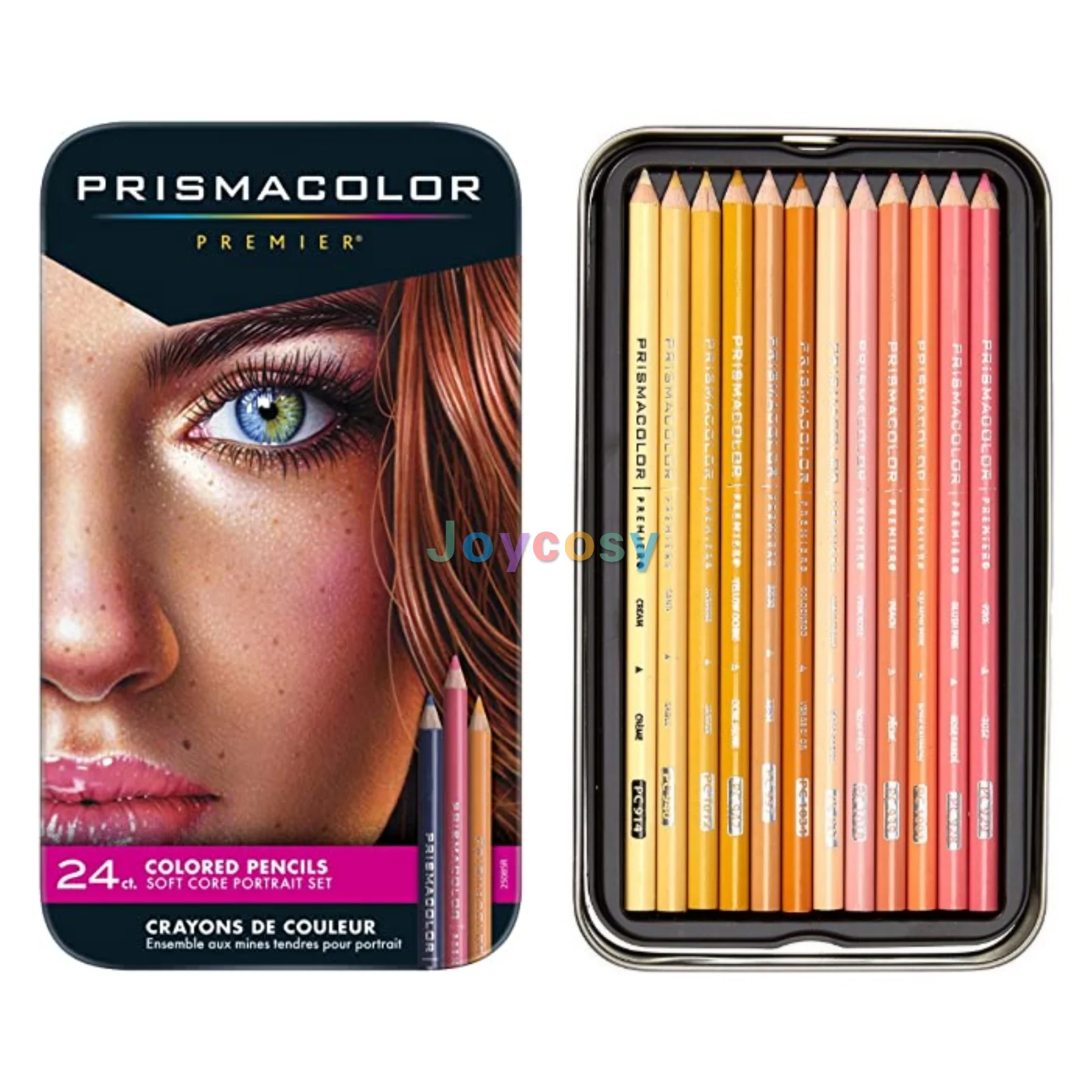The image is an advertisement for a Prismacolor colored pencil set, likely found in a catalog or on a website. The left-hand side of the image features the packaging, which is the front part of the tin that stores the pencils. The tin has a black background with "Prismacolor" written in white, beneath which is a rainbow line transitioning from blue to green, yellow, peach, magenta, and navy. Below this, "Premier" is written in yellow. A detailed colored pencil drawing of a woman's face is displayed on the lid, showing just her left eye adorned with mascara and eyeliner, along with noticeable freckles. Below the woman's face, "24 count colored pencils soft core portrait set" is printed in magenta, followed by "Crayon de Color" in a black banner, with translations in French and Spanish. On the right-hand side of the image, the inside of the pencil box is displayed, revealing the vibrant colored pencils neatly lined up. The pencils range in color from pale yellow to darker shades of yellow, pink, coral, and salmon pink. There is also a watermark across the image that says "July Cozy."